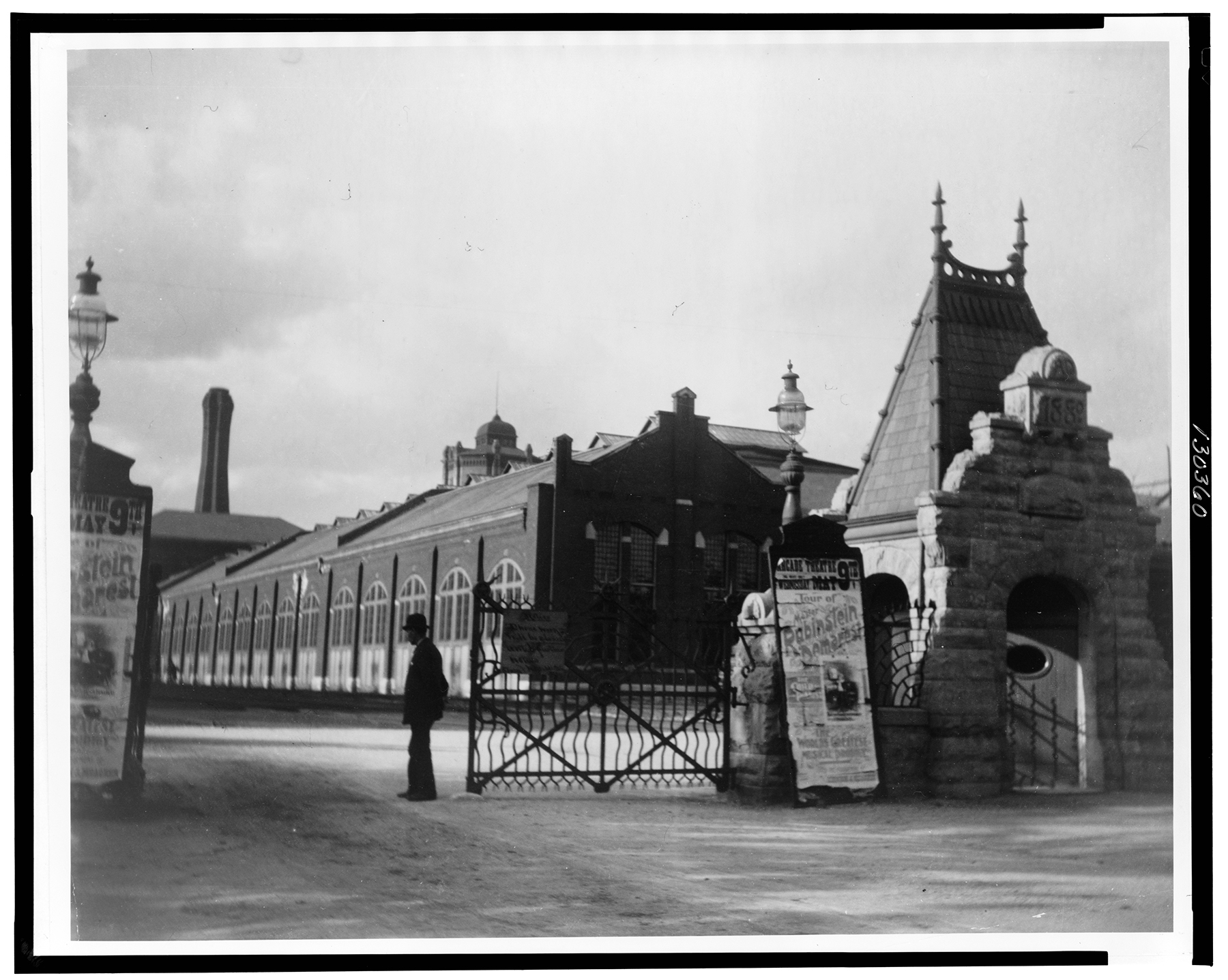The black and white photograph, framed with a thin black border and an inner white border, captures a vintage scene likely from the 1930s. Dominated by shades of gray and black, the image showcases a large, expansive building in the background, with numerous windows visible, possibly a pavilion for fairground events. In the foreground, a wrought iron fence or gate, partially open, stands prominently at the center, leading into what appears to be a large fairground area. To the left of the gate, a man dressed in a suit coat and top hat faces towards a streetlight post, which is also on the left side of the image. On the right side, there is a substantial brick structure with an arched opening, resembling a ticket booth area where tickets might be sold for events. Above this structure, a streetlight can also be seen in the background, adding depth to the scene. The ground beneath the elements is a consistent gray tone, and the sky above is a mixture of light gray and white, enhancing the vintage feel of the image.